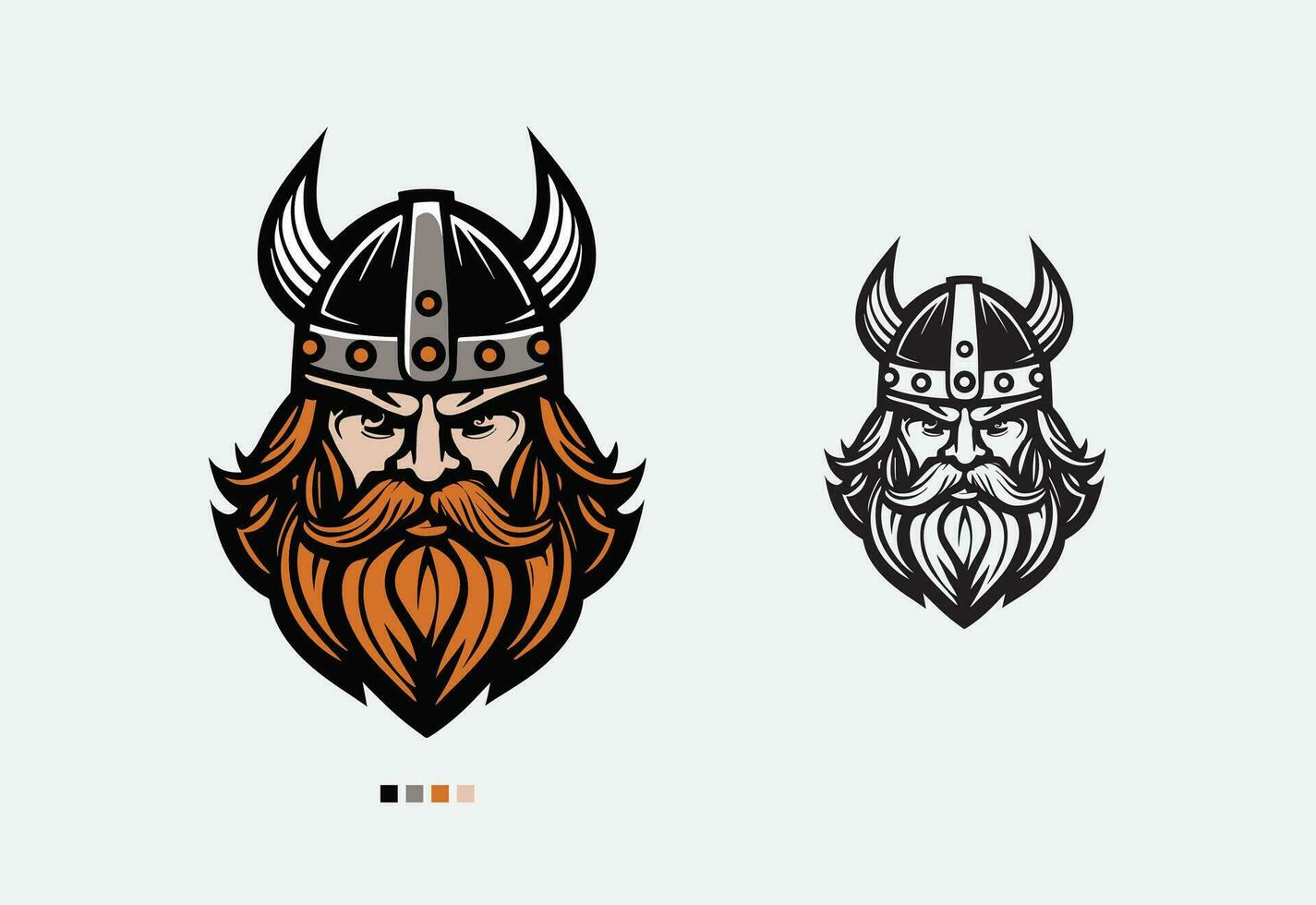This vivid, computer-generated landscape illustration showcases two strikingly similar Viking figures, positioned side by side. The left figure, portrayed in full color, is a stern, middle-aged Viking with a shaggy, golden-brown beard and mustache. He has an intense, menacing glare with furrowed brows, tiny eyes, and shaggy eyebrows. His traditional Viking helmet, adorned with two prominent horns, features a black center with silver straps and bolts, accented by orange beads. To the right, a slightly smaller, black-and-white replica of the Viking mirror reflects the same fierce expression and intricate helmet design. The black-and-white version resembles a tattoo design, accentuating its detailed and perfect form. This image appears to originate from a website offering customizable team logos, as indicated by the color scale beneath the larger Viking, which suggests the ability to alter his colors.